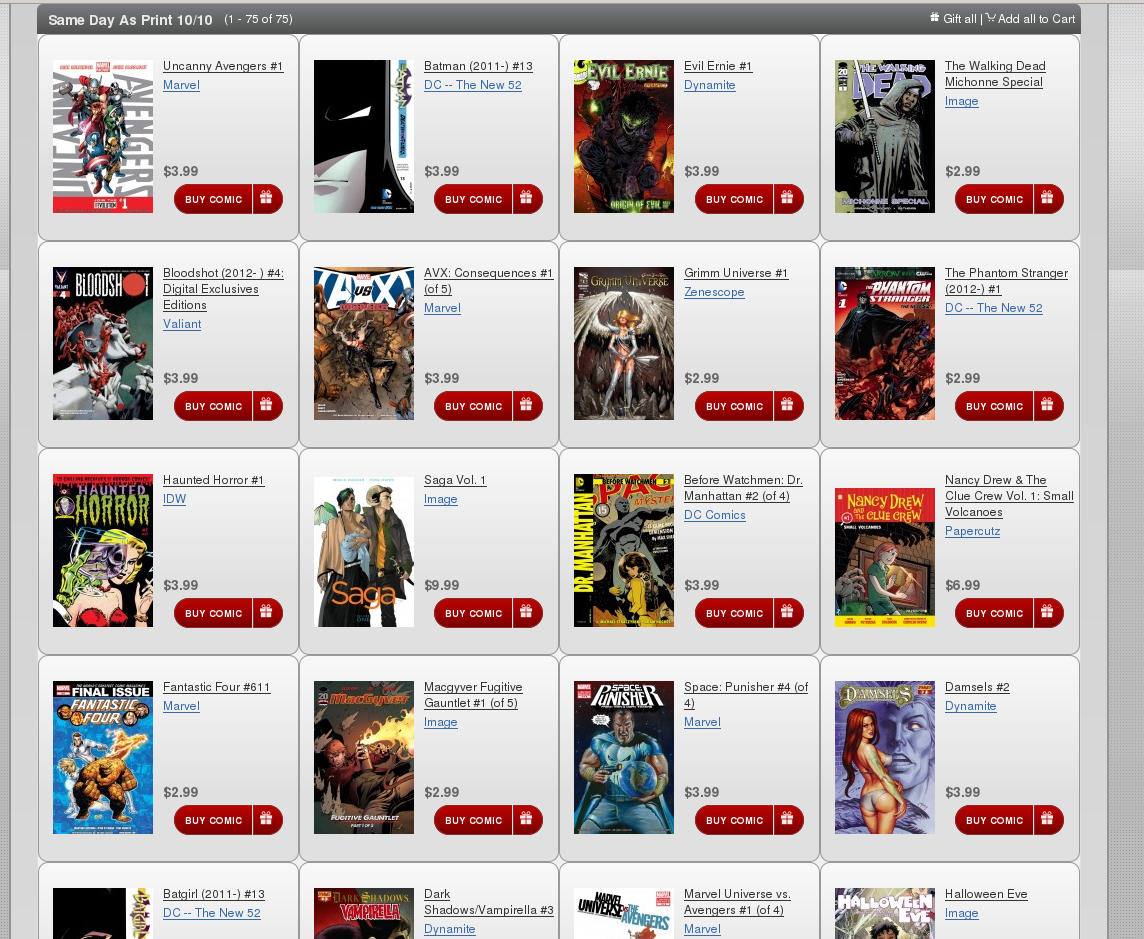This webpage is dedicated to the purchase of Marvel comic books. At the very top, there is a dark grey banner displaying the text "Same Day as Print 10/10," accompanied by a series of numbers on both the left and right corners. Below this, the layout is filled with comic book listings arranged in a grid format—four comic books across and four and a half rows down, with a glimpse of the fifth row. Each comic book is presented within a grey background box, featuring a picture of the cover on the left side. Adjacent to each image is a detailed description of the comic book, including its title, brief summary, and price. 

A red button labeled "Buy Comic" appears alongside each listing, providing a convenient option for purchasing. Additionally, a small gift box icon is present within each listing, indicating the availability of more details about the product, including its cost. Users can click on these elements to either buy the comic directly or to learn more about its content. The selection includes a variety of titles such as "Avengers," "Haunted Horror," and "MacGyver," among others, catering to diverse comic book interests.